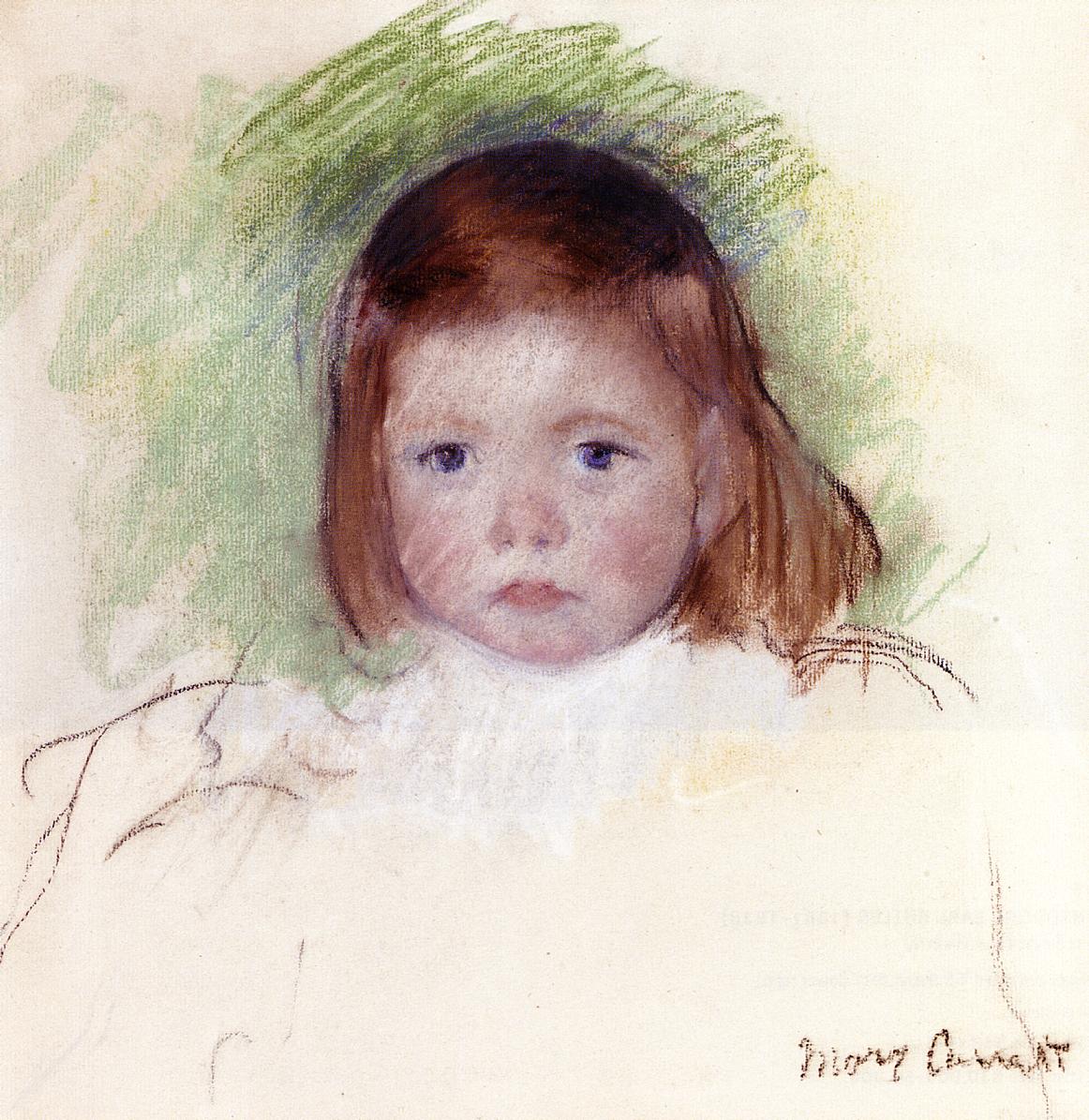This painting depicts a young girl with a somber expression, centered in a square, cream-colored background. She has red hair, cut square at the top and falling just below her ears, with dark brown eyebrows. Her face, which dominates the image, features full, pink cheeks and blue eyes that stare directly ahead, conveying a sullen demeanor. A distinct halo of green hues, ranging from light green to lime green, surrounds her head, extending from her shoulders upwards. Only the outlines of her shoulders are faintly visible. The artwork is signed by the artist, Mary C., in the bottom right corner. Light brown strokes add texture to the lower corners of the painting, enhancing its depth.